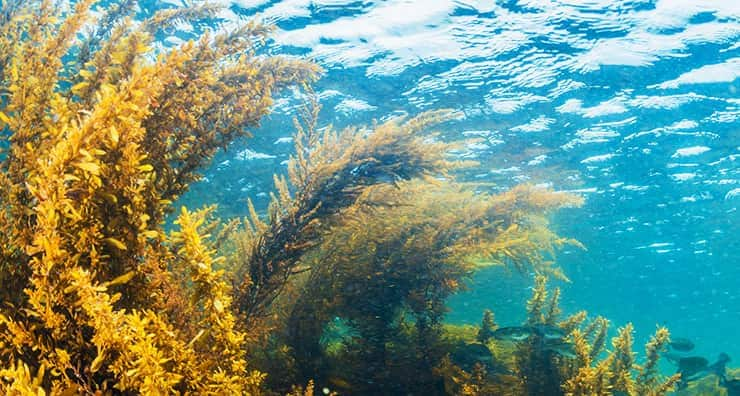This underwater photograph captures a serene aquatic scene with a clear view towards the water's surface, revealing ripples and white shimmering spots where the sunlight penetrates. The water is a vibrant light blue, creating a tranquil backdrop. Dominating the lower left corner and extending through the center of the image are varied species of algae and underwater plants. These plants, ranging in color from yellowish-golden to brownish-green, stand tall with stringy, lanky stems that arc gracefully to the right. Their leaves drape elegantly, providing substantial plant cover over the ocean floor. Amidst these plants, a group of around ten small, darkish-gray fish can be seen on the lower right side, swimming in and out of focus due to the underwater camera's slight blur. The overall image, with dimensions reminiscent of a high-definition TV, emphasizes the lush underwater vegetation and the serene, sun-dappled water above.